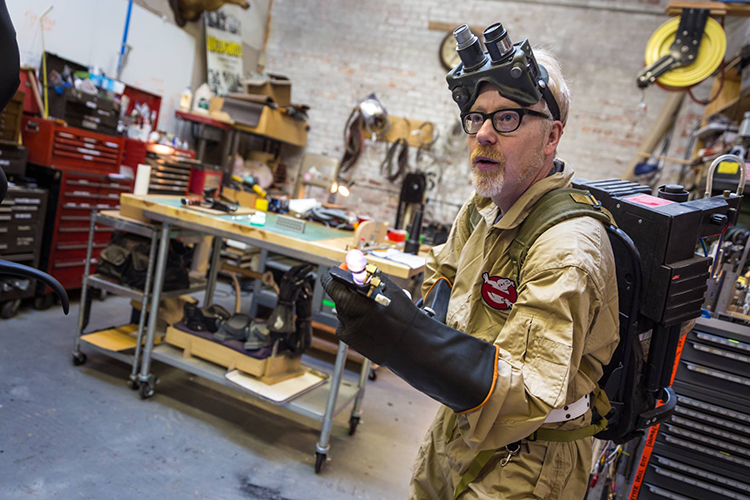A detailed caption for the image could be:

"In a well-organized workshop filled with various cabinets, a person is dressed in detailed Ghostbusters attire. The individual wears a tan jumpsuit paired with black rubber gloves. Strapped to their back is a proton pack, designed to capture ghosts, which is secured in a backpack fashion. In their hand, they hold a proton wand connected to the pack, essential for ghost containment. On their head, they sport ordinary black-rimmed glasses, but resting on their forehead are a specialized pair of binocular-like devices. The individual gazes upwards, exuding the aura of a dedicated ghost hunter. The workshop setting, with visible red cabinets to the left and a centrally located work table, suggests it is the place where they assembled their intricate ghostbusting gear and costume."